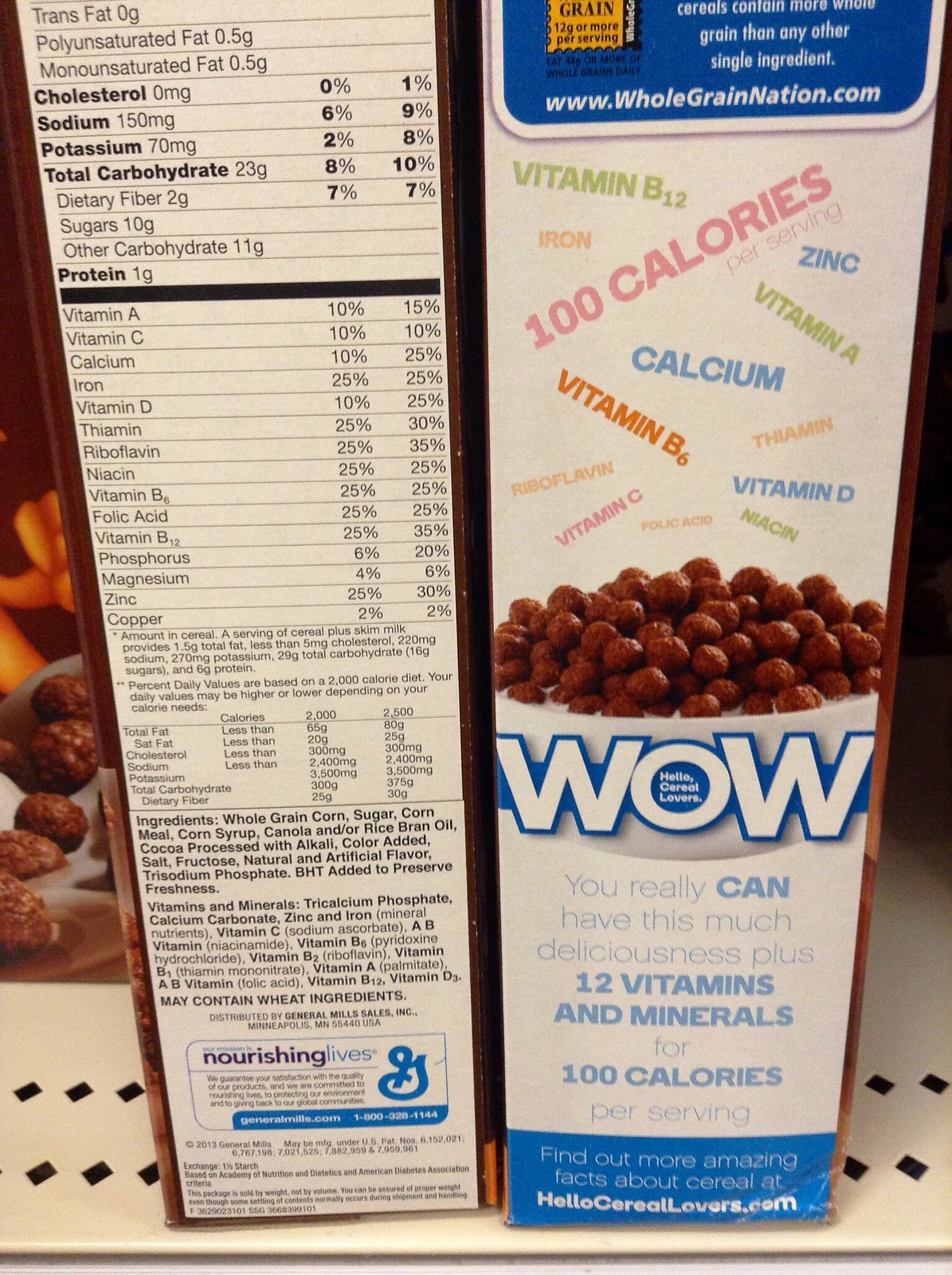The image showcases the side panels of whole grain cereal boxes displayed on a supermarket shelf. The leftmost box partially reveals a nutrition panel listing trans fat, polyunsaturated fat, monounsaturated fat, cholesterol, sodium, potassium, total carbohydrate, protein, and a comprehensive list of vitamins and minerals including Vitamin A, Vitamin C, Calcium, Iron, Vitamin D, Thiamine, Riboflavin, Niacin, Vitamin B6, Folic Acid, Vitamin B12, Phosphorus, Magnesium, Zinc, and Copper. Below the nutrition facts, the ingredients are detailed, featuring whole grain corn, sugar, corn meal, corn syrup, canola oil, and rice bran oil. At the bottom, the General Mills logo is shown, alongside a phrase promoting the cereal as a healthy option, "Nourishing Lives."

The rightmost box highlights additional features in a visually engaging format. At the top, the website www.wholegrainnation.com is visible, followed by a graphic depicting a bowl of chocolate cereal balls in a white bowl, likely Cocoa Puffs, with the word "WOW" prominently displayed above it. Surrounding the bowl are graphics listing the included vitamins and minerals such as Calcium, Vitamin B, Vitamin A, Zinc, 100 calories, Vitamin B12, Vitamin D, and Vitamin C. Below the bowl, a tagline reads, "Hello, cereal lovers," emphasizing the cereal's appeal and nutritional value, stating that one can enjoy "this much deliciousness plus 12 vitamins and minerals for just 100 calories per serving." Further details can be found at hellocereallovers.com. The background incorporates diamond-shaped cutouts, adding to the visual texture.